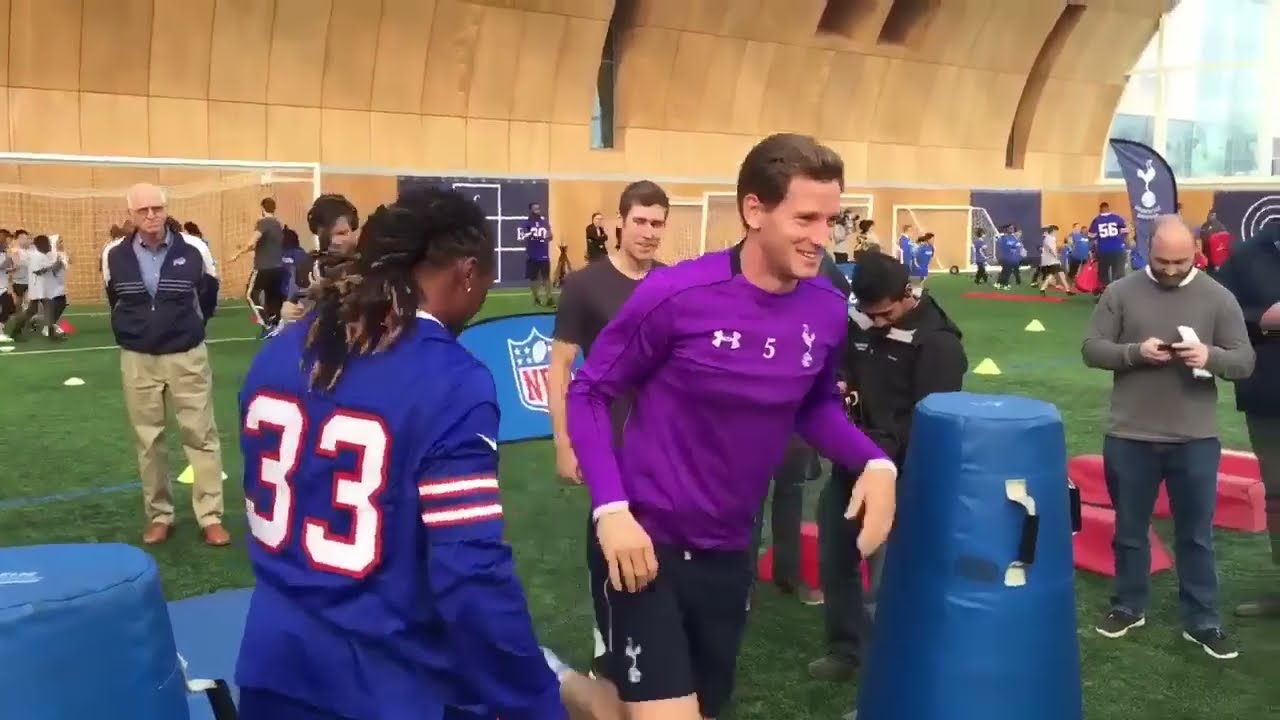The image depicts a football training camp, specifically an NFL-sanctioned event, likely intended for mentoring kids. The scene takes place in a facility with green AstroTurf, possibly an indoor practice center or stadium field, as indicated by the presence of soccer goals and a curved sandstone-colored wall in the background. Central to the image is a Caucasian gentleman with light brown hair, clad in a light purple, long-sleeved Under Armour shirt and black shorts. He appears to be running through an agility drill between two tall, blue foam pads with handles. Near him, an African-American person with long dreadlocks pulled back, wearing a purple long-sleeved jersey marked with the number 33 and white bicep stripes, is also engaged in the activity. Scattered around them are several onlookers, some with cameras and clipboards—potentially coaches, reporters, or spectators—all smiling, implying a lighthearted practice atmosphere. In the background, various players and groups of children are visible, underscoring the camp's youth-oriented focus. An NFL poster further cements the professional affiliation of the event.